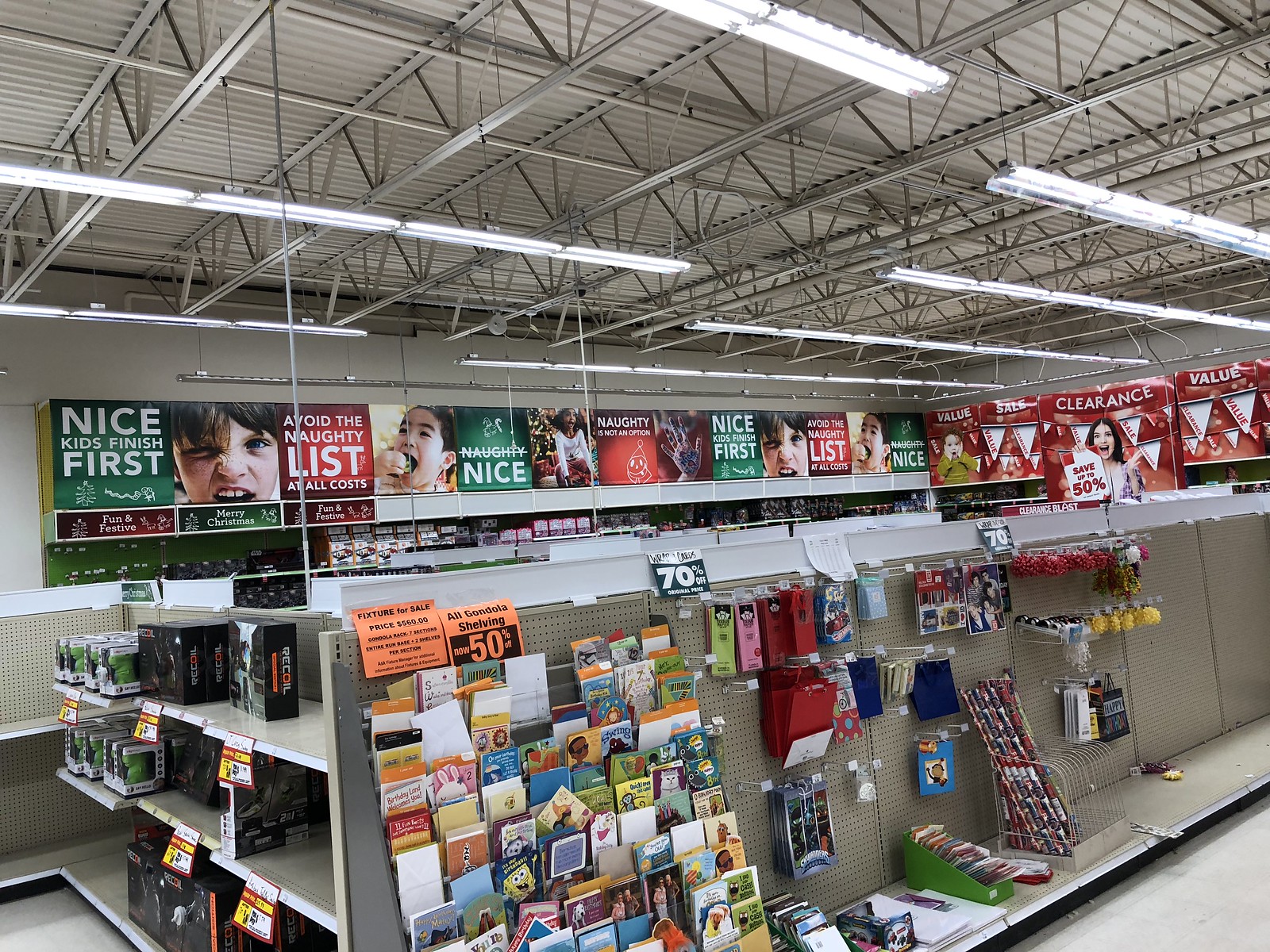The image depicts a spacious aisle inside a store, possibly a grocery or general merchandise store, characterized by its industrial aesthetic. The ceiling, approximately 20 feet high, features corrugated metal panels and gray beams, with long, tubular fluorescent lights hanging down to brightly illuminate the scene. The walls and shelves are also a matching gray, contributing to the utilitarian feel of the environment.

Central to the aisle is a somewhat sparse display of multicolored greeting cards in yellow, white, and orange, alongside gift bags, hinting at preparations for a festive occasion, possibly Christmas. Above this display are orange signs with black text, indicating fixture sales and 50% discounts on gondola shelving. Numerous sale signs clutter the scene, including a black box boldly proclaiming "Now 50% off" in striking orange text.

In the background, a variety of vibrant banners and advertisements stretch across the top of the scene, filling the upper space. These signs, rendered in green and red with white text, revolve around a Christmas theme, with messages like "Nice kids finish first" and "Avoid the naughty list at all costs." These ads feature images of children with varying expressions, from a sneering boy to a smiling child. Additional messages include "Naughty" and "Nice," with festive elements subtly integrated. Further along, a sign in bold declares "Clearance," accompanied by a picture of a woman with dark hair, underneath another offer to "Save up to 50%."

Overall, the scene exudes a transitional atmosphere, possibly suggesting the aisle is being prepped for an upcoming seasonal sale, with empty spaces and partially stocked shelves hinting at ongoing arrangements.